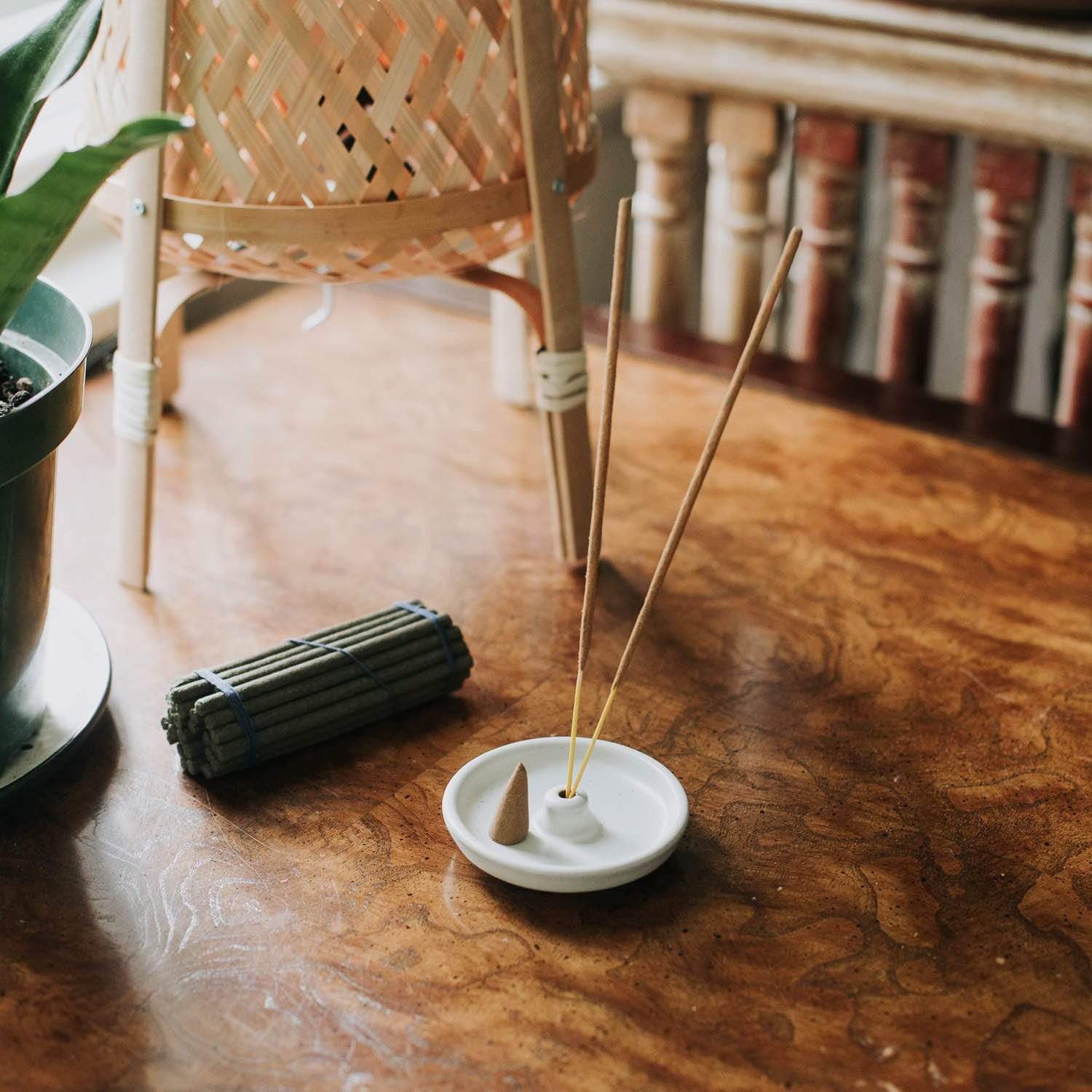The image depicts a wooden desk with several objects arranged on top. Dominating the scene is a small, white, ceramic dish sitting in the center, which functions as an incense holder. The holder contains two unlit incense sticks and one unlit incense cone. Adjacent to the dish is a bundle of green sticks, thicker and shorter than the incense sticks, tied together with rubber bands. To the left is a green plant in a green pot, placed in a matching saucer, with long, lush leaves extending beyond the frame. Additionally, there is a distinctive wicker lamp on the desk, featuring an intricate woven pattern that suggests it could also be mistaken for a planter. In the background, part of a railing with columns is visible, adding to the domestic ambiance of the scene.